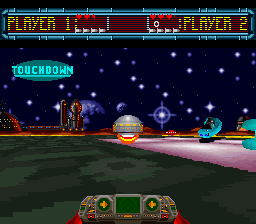In this captivating screenshot from a video game, the upper section features a brownish-red box with yellow letters displaying "Player One," accompanied by a small adjacent box, and another box showing "Player Two" with a score of zero. The background is an enchanting dark blue sky peppered with white stars. Prominently, the word "Touchdown" is displayed in green with a corresponding green circle around it. The scene showcases a couple of space-themed characters standing on a narrow walkway. Various elements are scattered around, including a vibrant star, a small vehicle, and a stretch of road with a gray round object resting on it. In the foreground, there’s a detailed visual of a game controller being grasped by someone's hands, adding an immersive touch to the gameplay experience.